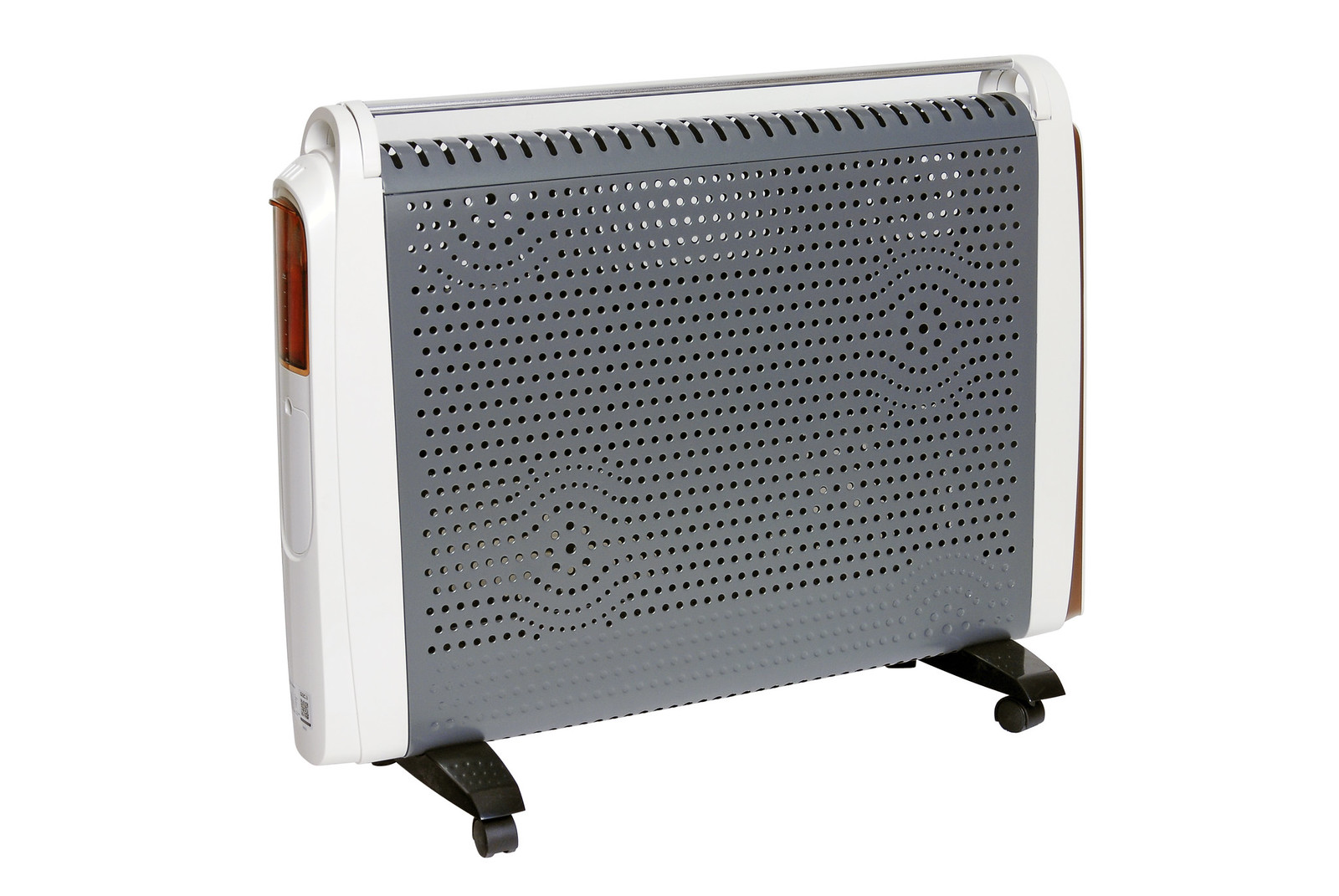This image features a portable heater with a distinct design. The heater's frame is predominantly white, with a central gray grid where the air flows out. This grid section is perforated with small holes for ventilation. Positioned at the top of the heater are additional vents for optimized airflow. A white handle is integrated at the top, allowing for easy portability. Notably, the heater includes two red indicator lights: a smaller one on the left side and a larger one on the right. The larger light might indicate whether the heater is on or off. At the base, the heater is supported by four black wheels, which are reinforced with black supports. There is also a small sticker featuring a barcode located at the bottom left corner, adding to its functional design details.